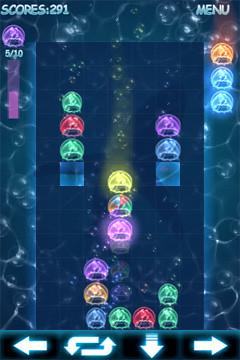In the top left corner, the image displays a score labeled "291" adjacent to the menu. Encircling the border are numerous bubbly visual elements, giving a sparkly, effervescent feel. Situated beneath a 5x10 grid, a prominent purple circle is accompanied by a purple bar. To the right, an arrangement includes an orange circle followed by two blue circles. The center of the image features a cascade of various colored circles—green, red, yellow, blue, rainbow-hued, purple, and blue—alongside a singular blue square. At the heart of this scene are three central elements colored purple, orange, and blue respectively. Below these, there is a sequence that starts with a green circle followed by a red circle and then two stacked green circles. In the bottom left corner, directional arrows guide attention: one points left, another loops upwards and to the right, one directs downward, and the last points to the right.